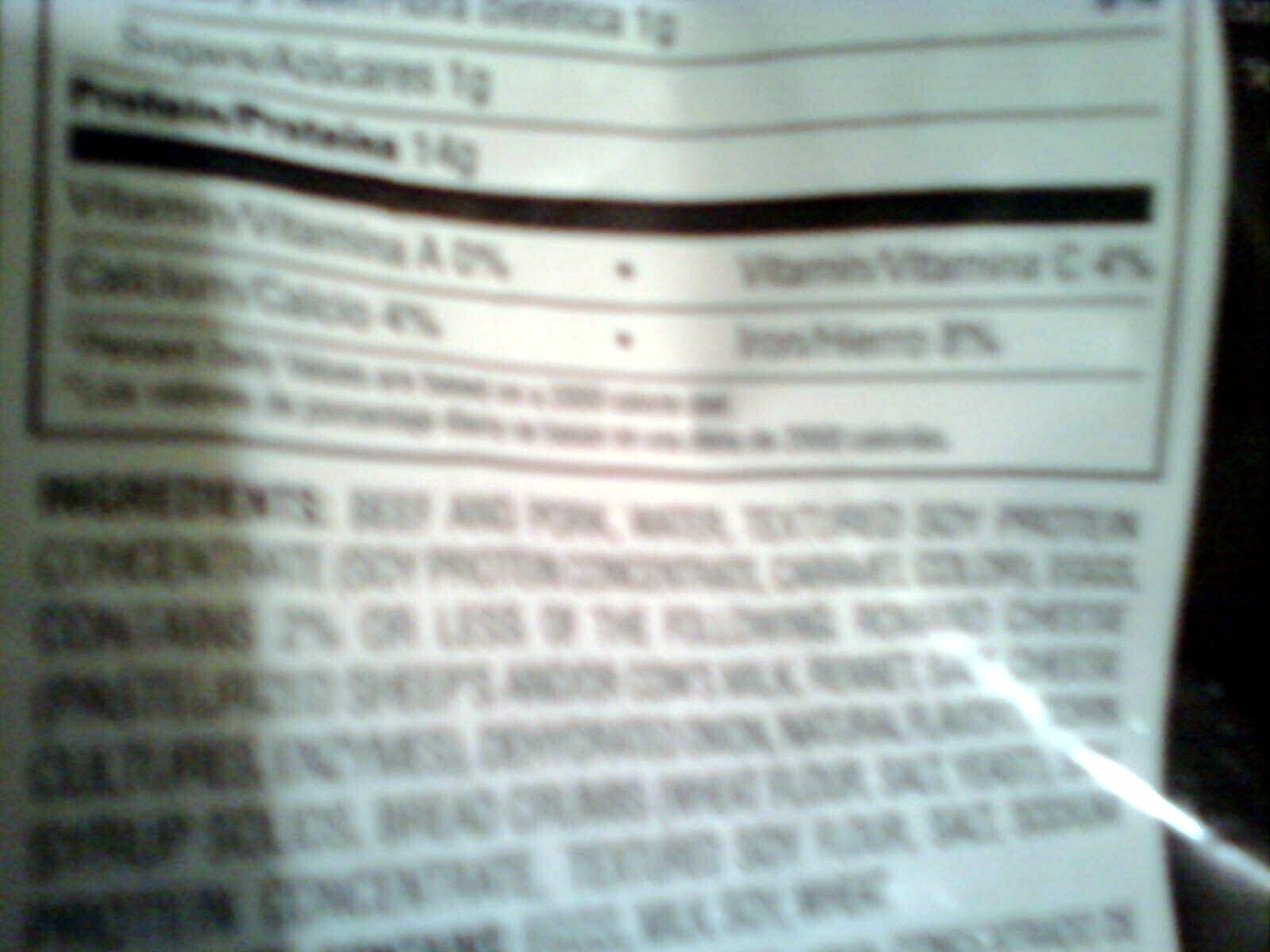This is an extremely blurry photograph of what appears to be the nutrition and ingredients label on the back of a food item package. The white label with black text is difficult to read due to the blurriness, strange angle, and light reflection on the plastic bag, suggesting the photo was taken indoors. Despite the poor quality, some information is partially discernible: it lists 1 gram of sugar, 14 grams of protein, zero percent Vitamin A, four percent Vitamin C, and conflicting reports of zero or four percent calcium. The rest of the nutritional facts and ingredients are unreadable due to the blurriness and the awkward angle at which the photo was taken. The packaging of the product appears to be black or dark-colored.